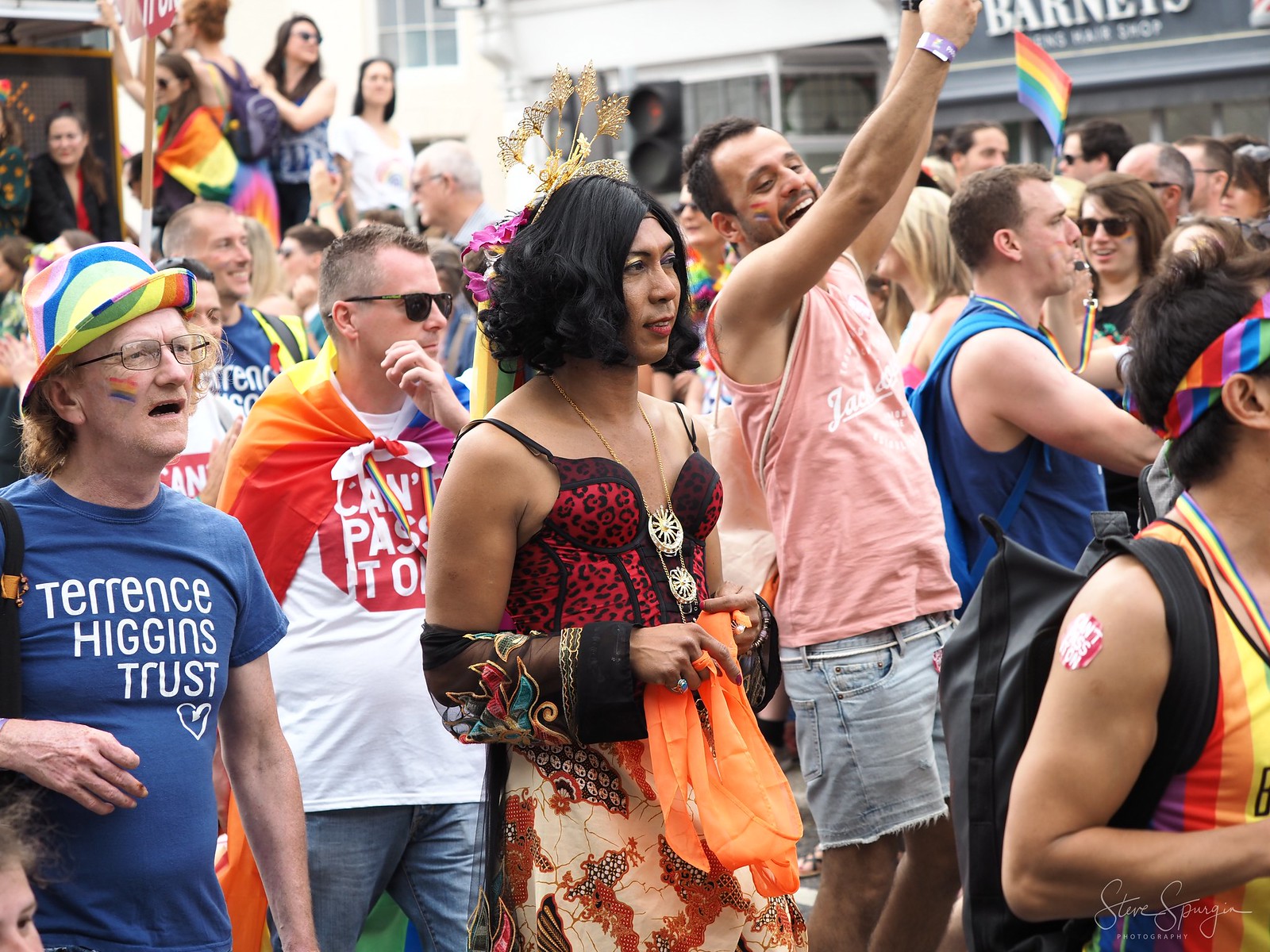The image captures a vibrant and bustling urban environment, likely downtown, showcasing a large crowd of people attending a gay pride parade. The crowd is adorned in rainbow-colored clothing, with many draping and waving pride flags. In the center of the frame, an individual with long, black hair—likely a wig—is seen wearing a leopard-print bra-like top with spaghetti straps and a dress. To the left of this person, a man in a blue short sleeve shirt with white text stands out. In the bottom left corner, an elderly man with glasses is seen wearing a purple shirt that reads "Terrence Higgins Trust," topped with a rainbow fedora hat and a small rainbow flag painted on his right cheek. Scanning further right, a man in a light peach-colored tank top and faded blue jean cutoffs energetically raises his hands. The background reveals multiple storefronts and a multi-story building, further highlighting the urban setting of this lively LGBT pride event.